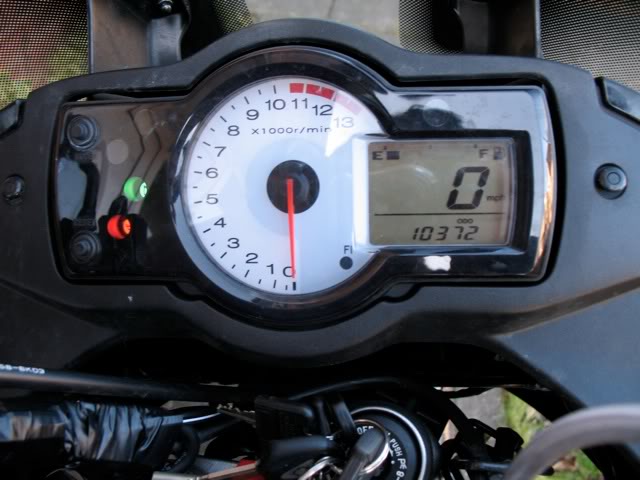This close-up photograph captures the intricacies of a motorcycle dashboard, highlighting the speedometer and tachometer with exceptional clarity. The dashboard features an analog tachometer with a white face contrasted by black numerals and ticks, making the readings easily legible. The tachometer’s numbers range from 1 to 13, signifying the engine's revolutions per minute, with the needle resting just below the 1 mark at 0 RPM. A red zone starts from 11, indicating the maximum safe engine speed. To the right of the tachometer, a digital display relays essential information: the vehicle is at a standstill, showing 0 miles per hour for speed, and the odometer reads 103.72 miles. Additionally, a horizontal bar at the bottom of the digital display represents the fuel gauge, which is currently at the halfway mark. On the left side of the dashboard, various indicator lights are visible, further adding to the informative yet aesthetic design of the motorcycle's control center. The entire assembly is encased in a sleek black housing, emphasizing both functionality and style.